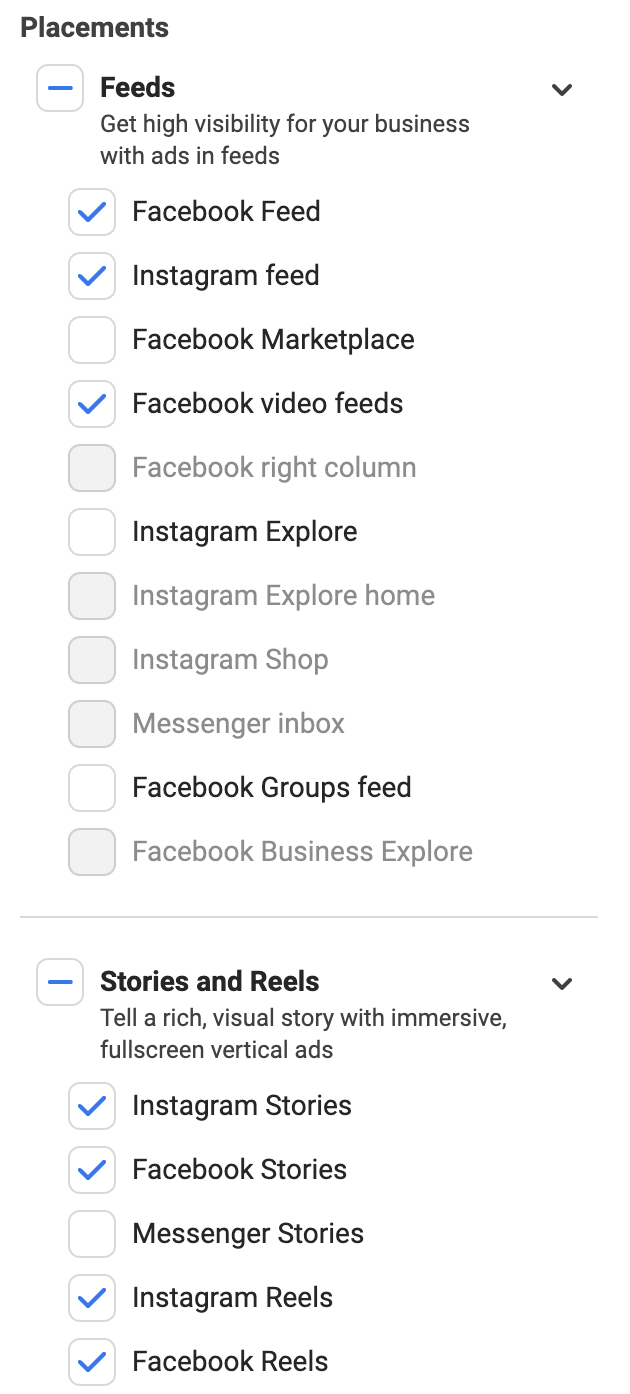Here’s a detailed and cleaned-up version of the provided voice caption:

---

This screenshot displays various advertising placements and feeds on a white background, each associated with a checkbox indicating their status. Below the section titled "Get high visibility for your business with ads and feeds," several placements are listed with their respective statuses:

- Facebook Feed: Checked
- Instagram Feed: Checked
- Facebook Marketplace: Unchecked (white box)
- Facebook Video Feeds: Checked
- Facebook Right Column: Unchecked (gray box)
- Instagram Explore: Unchecked (white box)
- Instagram Explore Home: Unchecked (gray box)
- Instagram Shop: Unchecked (gray box)
- Messenger Inbox: Unchecked (gray box)
- Facebook Groups Feed: Unchecked (white box)
- Facebook Business Explorer: Unchecked (gray box)

The text "Facebook Feed," "Instagram Feed," "Facebook Marketplace," "Facebook Video Feeds," "Instagram Explore," and "Facebook Groups Feed" appear in bold to emphasize their importance.

Further down, in the section dedicated to stories and reels, it states, "Tell a rich visual story with immersive full-screen vertical ads." The following placements are listed with their respective statuses:

- Instagram Stories: Checked
- Facebook Stories: Checked
- Messenger Stories: Unchecked